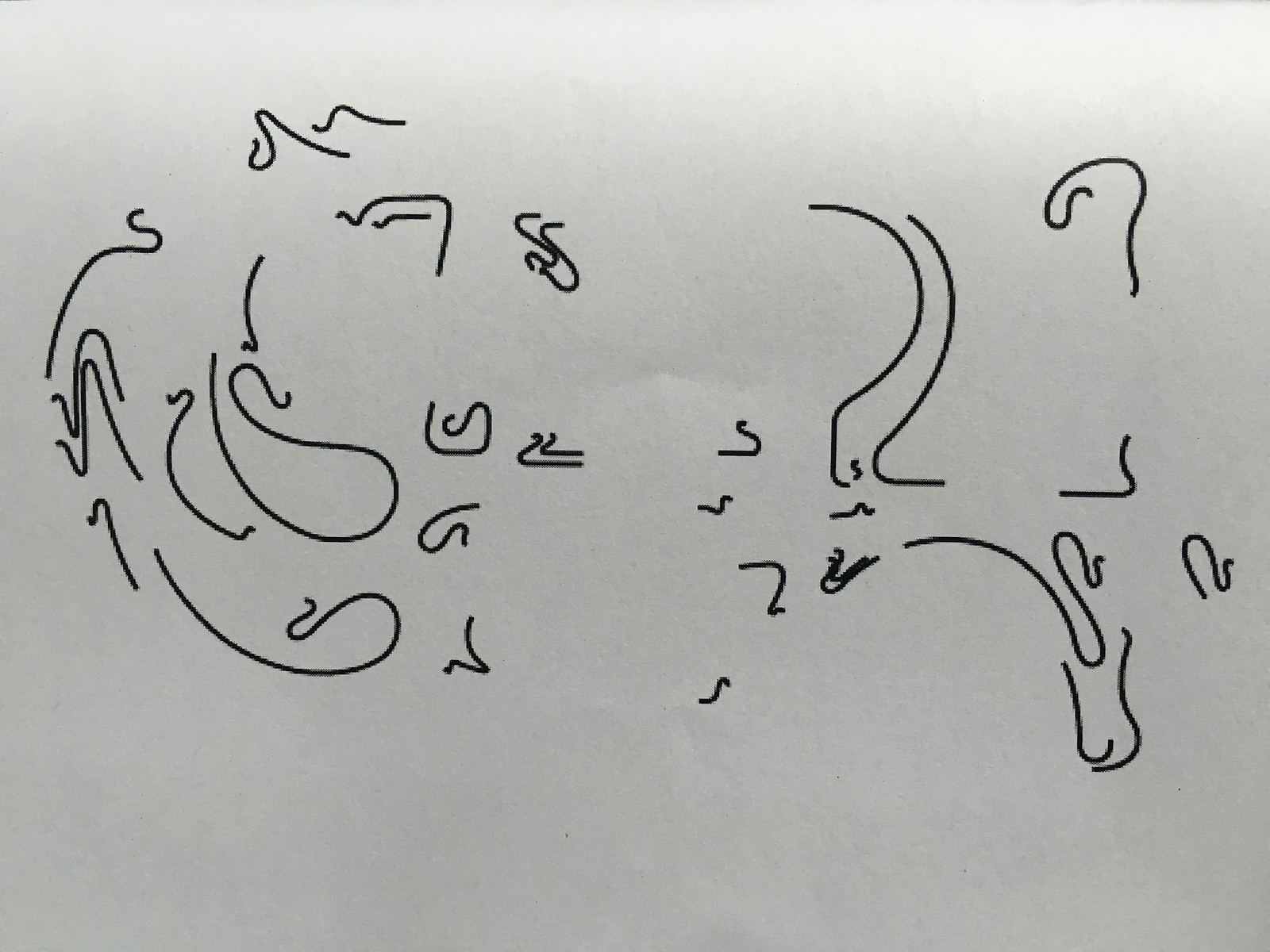This image features a collection of black squiggles on a white background resembling an actual piece of paper. The squiggles, slightly pixelated, suggest they are digitally drawn. The large, curvy lines dominate the composition, with some on the left forming hook-like shapes reminiscent of hangers. A few curves resemble the silhouette of a duck. Interspersed among these are smaller squiggles, some appearing as check marks, others as tiny earring hooks. The right side showcases lines shaped like backward C's, merging to form a machete-like figure, alongside more earring hook shapes that curve back and outward.